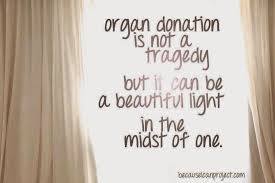The image captures an inspirational scene promoting organ donation. A beige curtain backdrop frames a sign with the quote, "Organ donation is not a tragedy, but it can be a beautiful light in the midst of one," written in an elegant, script-like font in brownish-gold lettering. This poignant message is illuminated by an overhead light that brightens the center of the scene, giving it a hopeful and uplifting atmosphere. The photograph seems to be from an event, possibly a gala or fundraiser focused on organ donation. The curtains are well-lit, enhancing the overall serene and encouraging mood of the setting. There is text at the bottom, possibly a website, though it remains unreadable.